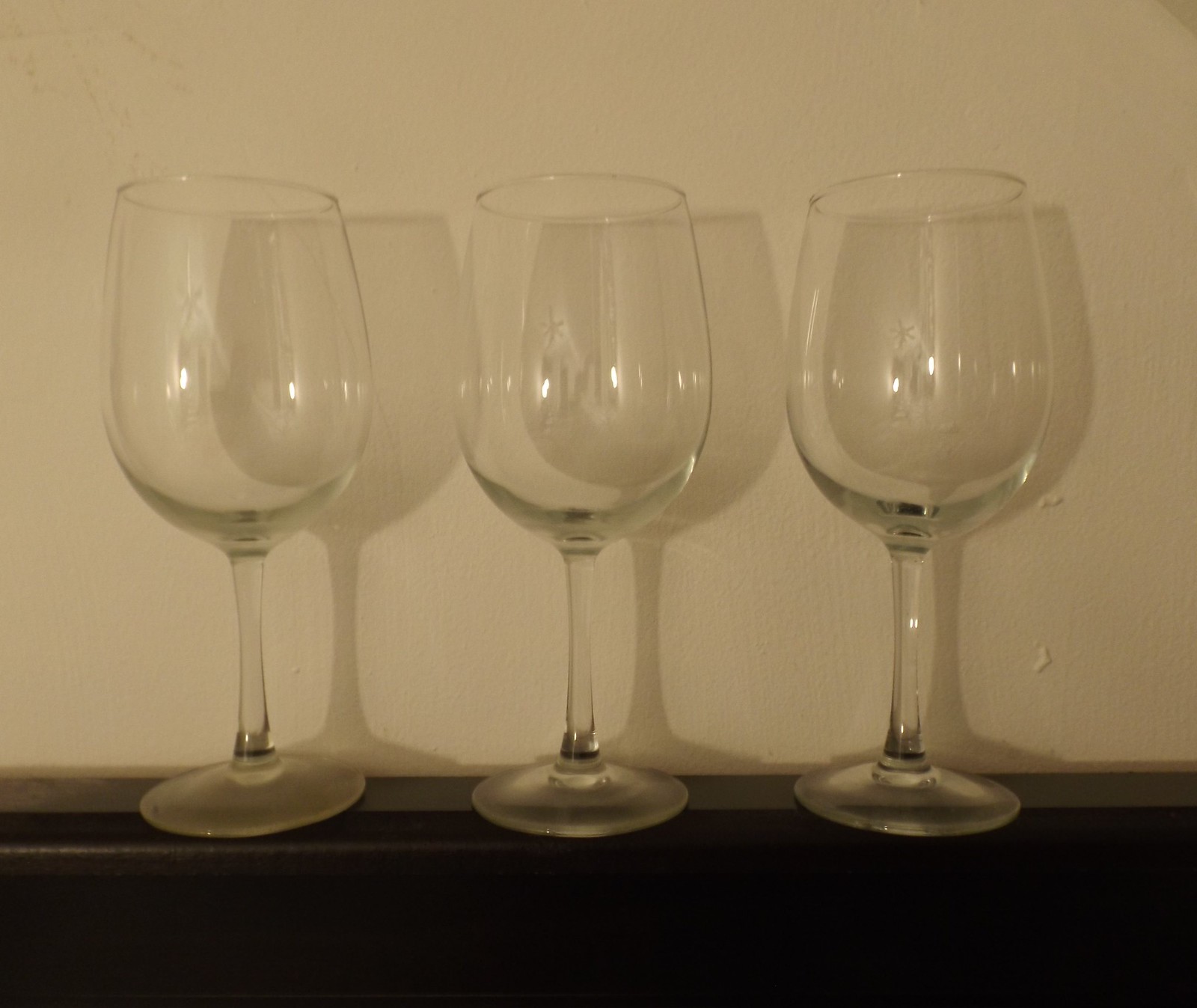This square-shaped, dimly-lit photograph captures three identical, clear wine glasses arranged side-by-side. They are positioned on a flat, dark brown wooden surface, which could be a table or a ledge. The glasses, featuring thin stems and flat bases, are prominently centered in the image. Each of these empty wine glasses reflects a ceiling fan and light, and possibly parts of a hallway. Behind the glasses, their shadows are cast onto an off-white wall. Notably, on the right-hand side of this wall, near the rightmost wine glass, there are some indentations or bumps, giving the wall’s texture a slightly irregular appearance.